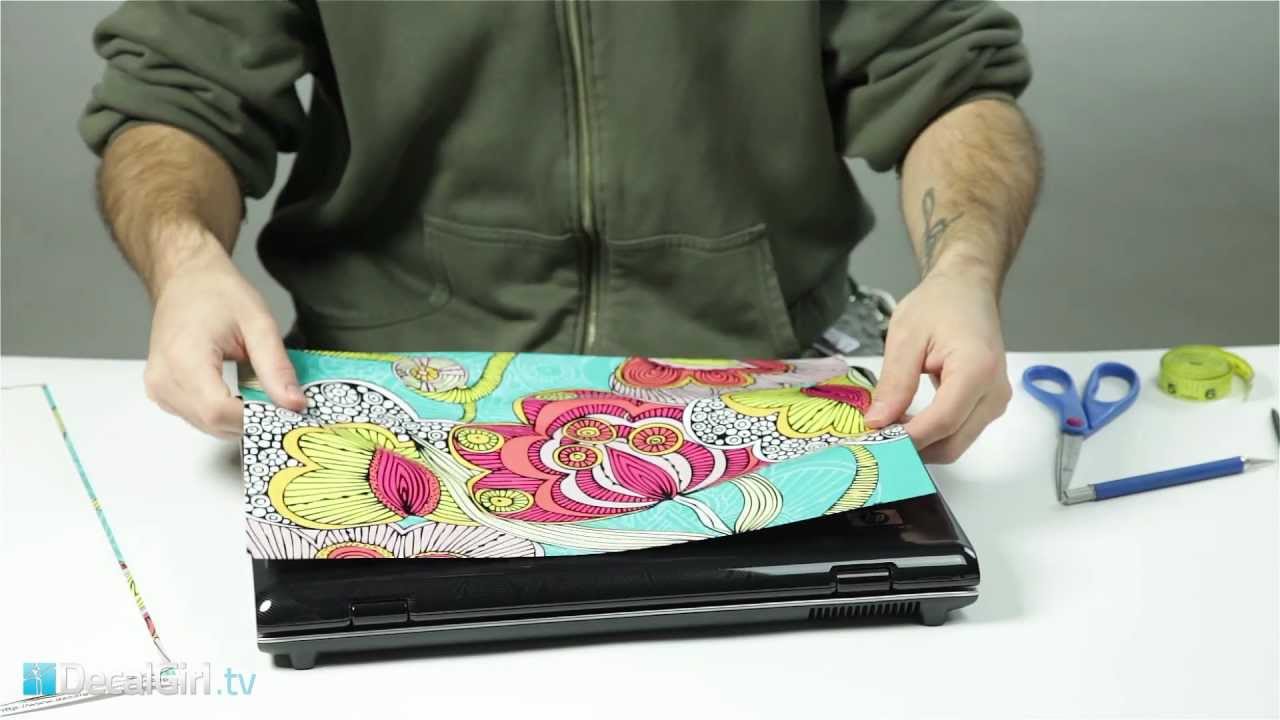The image features a man wearing an olive green, zipped-up jacket, visible only from the lower torso down. He is fair-skinned with dark hair on his forearms and a black tattoo on his left forearm. The man is standing over a white table with a black laptop on it. He is carefully placing a piece of detailed artwork on top of the laptop, possibly to personalize it. The artwork includes various flowers: a yellow flower with a pink center, a pink flower with yellow patterns, and black and white linear designs on a turquoise background. Surrounding the man are blue-handled scissors, a blue pen, and a yellow measuring tape. The setting appears to involve some kind of machine, possibly for creating decals, as indicated by the partially visible "designgirl.tv" logo in the bottom corner. The background is gray, providing a neutral backdrop to the scene.